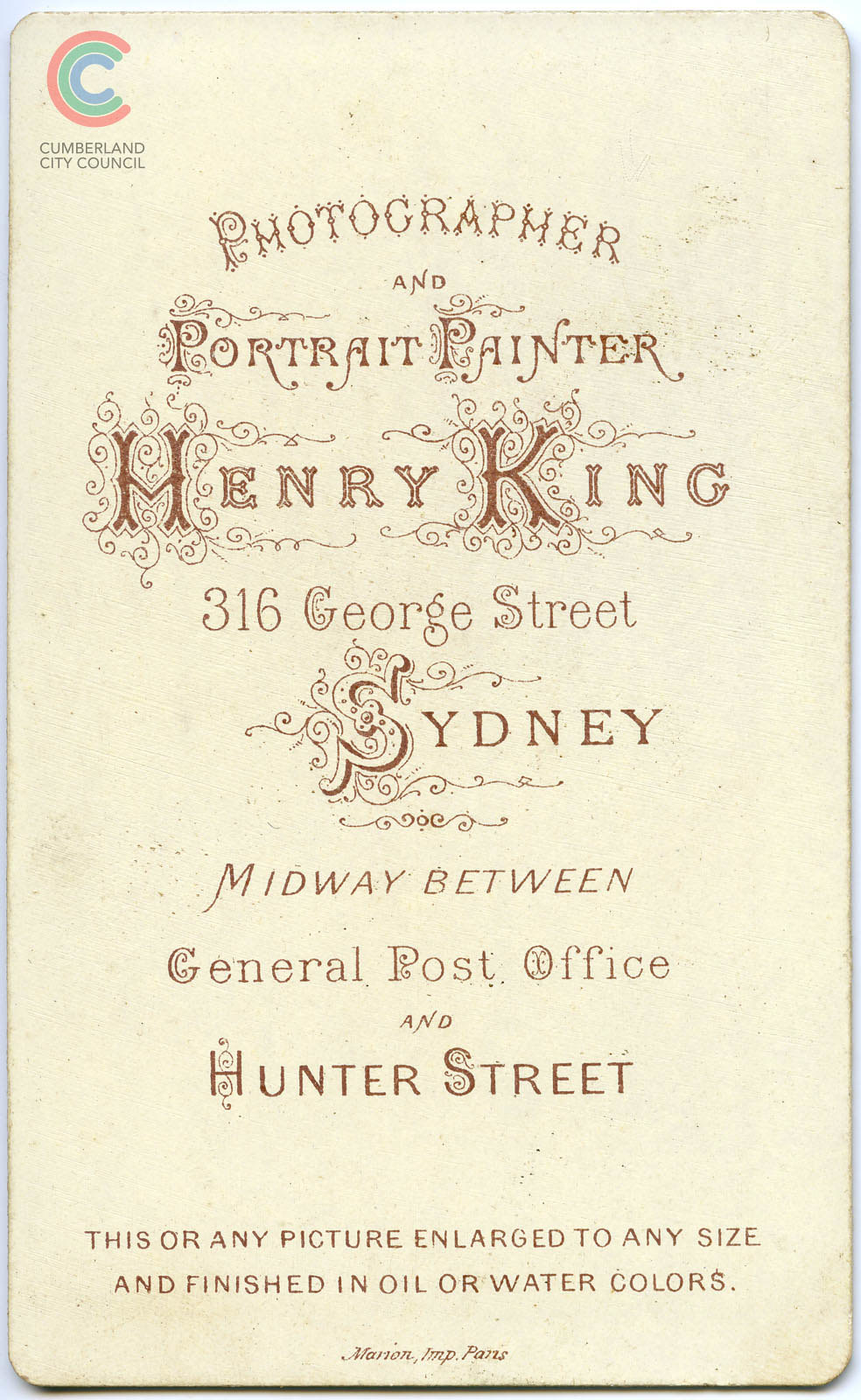The image features an ornate advertisement that appears to be either a vintage sign or the cover of a book. The background is a grainy, light beige with a subtle pink tint, complementing the predominantly brownish-red text that decorates the surface. In the top left corner, there's a logo composed of three concentric C's in blue, green, and red. Beneath this logo is a small line of black text that reads "Cumberland City Council."

The main portion of the text is centrally aligned and employs a variety of fonts, ranging from simple to very ornate. The text at the center begins with "Photographer and Portrait Painter Henry King," prominently featured in elegant, capitalized letters, with the initials "H" and "K" notably larger and highly stylized. Directly below this, the text provides the address: "316 George Street, Sydney, midway between General Post Office and Hunter Street."

Further down, in regular capital letters, it states, "This or any picture enlarged to any size and finished in oil or watercolor." At the very bottom of the advertisement, in small script that is somewhat difficult to read, it appears to say "Marion Imp. Paris," suggesting perhaps the maker or origin of the ornate design.

Overall, the presentation is highly detailed and ornate, with a clear emphasis on creating a vintage, artistic aesthetic through the use of varied fonts and careful text placement.